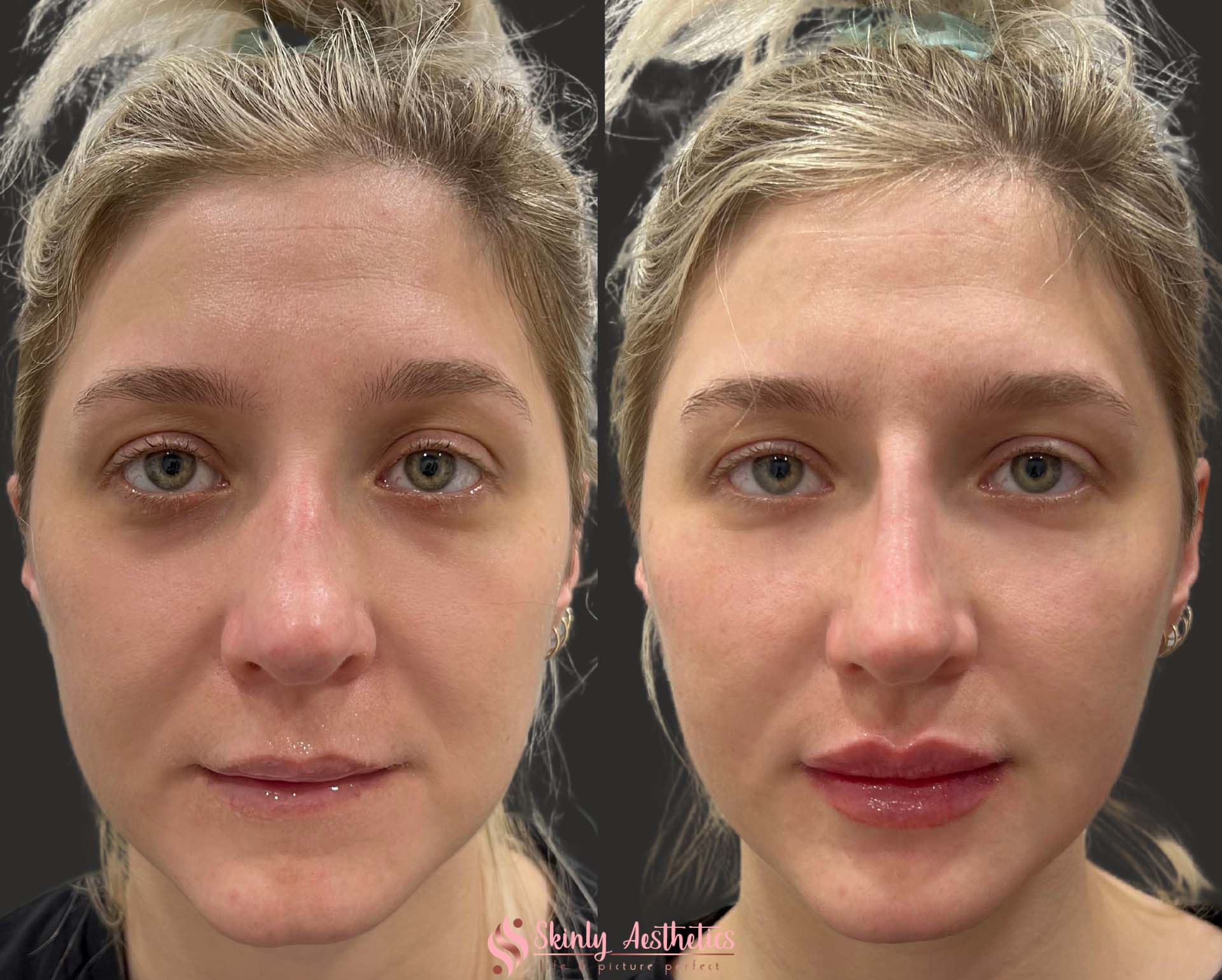This image is a detailed before-and-after advertisement featured by Skinly Aesthetics, set against a darker grey to black split-screen background. On the left side, we see a close-up of a blonde woman with hazel-green eyes, exhibiting a natural look with thin lips, dark circles under her eyes, a few forehead lines, and some blemishes on her chin. Her hair, less styled, frames a more bulbous nose and she isn’t wearing makeup. On the right side, the same woman appears post-treatment, with noticeable enhancements: her lips are fuller, the dark circles underneath her eyes are diminished, and her nose looks more refined and less bulbous, suggesting potential makeup or cosmetic procedure. The woman's hair is neatly styled, swept back, and subtle makeup highlights a dramatically improved and polished appearance. In this second photo, her more pronounced hoop earrings are also visible. At the bottom of the image, the text reads "Skinly Aesthetics, Picture Perfect," underscoring the transformative impact of their aesthetic services.